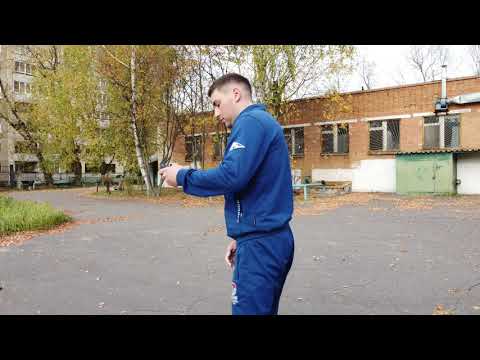The image features a white man in his 20s or 30s standing in the center of a gray parking lot, looking to his left and holding an unidentified device in his left hand. He is dressed in a dark blue tracksuit with white emblems on the sleeves and pants, and has short brown hair. Behind him lies a long, muted orange brick building with several uniform windows covered by chain-link fencing. A small green access door or box is visible on the building's side, surrounded by a larger green area next to a white wall. A mix of scraggly trees, some leafless and others with sparse green or dried leaves, is scattered around. To the left, a taller building, possibly an apartment complex with balconies, is partially obscured by the trees. The ground is strewn with fallen leaves, and the sky above is a cloudy blue, suggesting it is fall. The image appears to be a still from a video, evident by the black bars at the top and bottom.